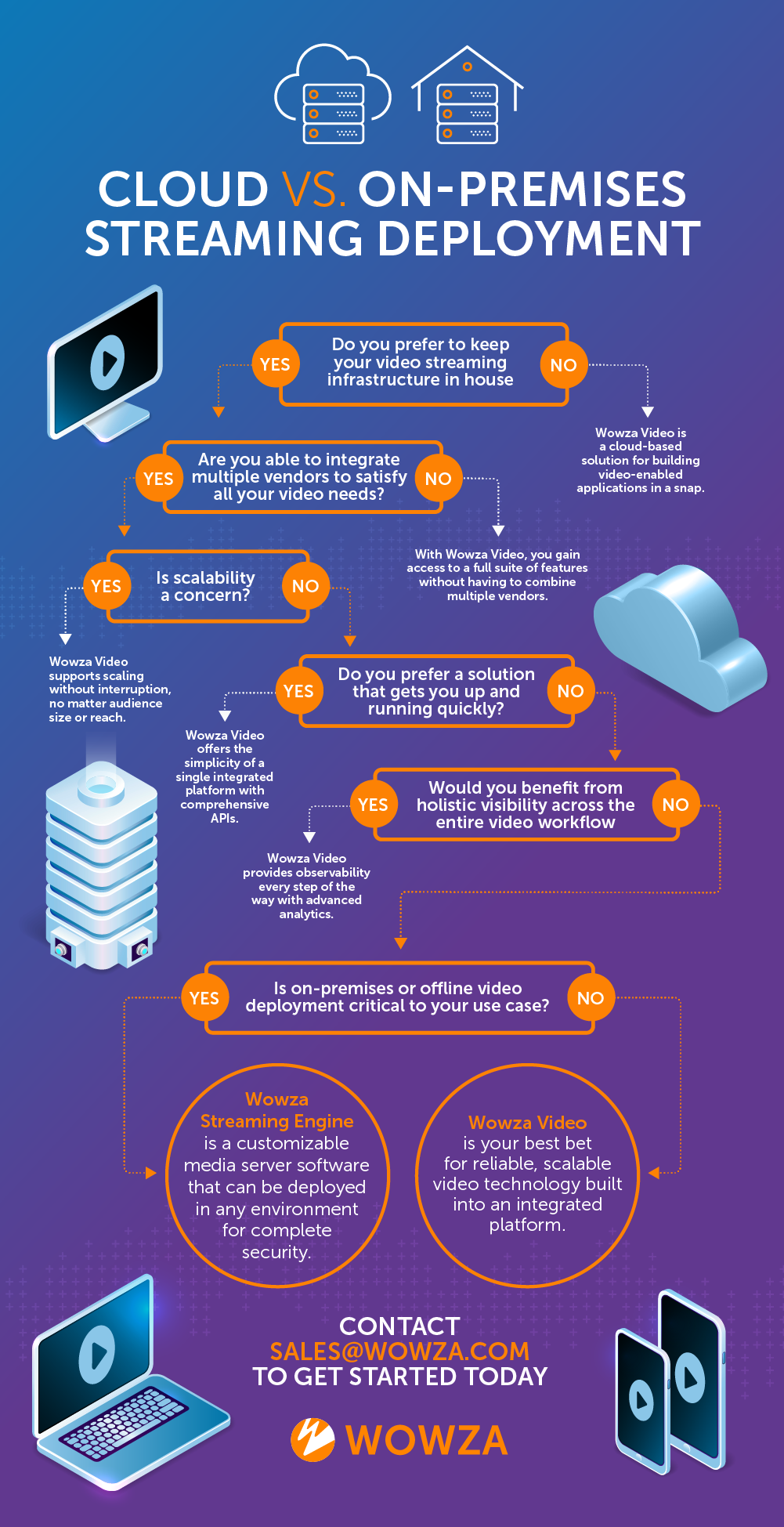This vertical advertisement, set against a gradient background transitioning from dark blue at the top to dark purple at the bottom, compares cloud-based and on-premises streaming deployment. At the top, the header "Cloud vs. On-Premises Streaming Deployment" is displayed, accompanied by two sets of images: a cloud with three computer boxes on the left, and a house with three computer boxes on the right. Below this, a detailed flowchart guides the viewer through a series of questions and decision points in white text, highlighted with orange boxes.

The flowchart begins with "Do you prefer to keep your video streaming infrastructure in-house?" If the answer is "No," it leads to the statement "Wowza Video is a cloud-based solution for building video-enabled applications in a snap." If "Yes," it progresses to "Are you able to integrate multiple vendors to satisfy all your video needs?" Answering "No," continues with, "With Wowza Video you gain access to a full suite of features without having to combine multiple vendors." Answering "Yes," advances to "Is scalability a concern?" If "Yes," it states, "Wowza Video supports scaling without interruption no matter the audience size or reach." If "No," it moves to "Do you prefer a solution that gets you up and running quickly?" If "Yes," it says, "Wowza Video offers the simplicity of a single integrated platform with comprehensive APIs."

Following this, "Would you benefit from holistic visibility across the entire video workflow?" If "Yes," it declares, "Wowza Video provides observability every step of the way with advanced analytics." If "No," it asks, "Is on-premises or offline video deployment critical to your use case?" Answering "Yes," leads to, "Wowza Streaming Engine is customizable media service software that can be deployed in any environment for complete security." All these paths and boxes are designed to guide users toward the optimal Wowza solution based on their needs.

At the bottom, the advertisement urges viewers to "Contact sales@wowza.com to get started today," with a Wowza logo and images including a computer monitor, a laptop, and two tablets, emphasizing the flexibility and comprehensive nature of Wowza's offerings.